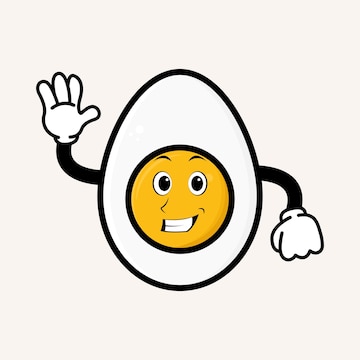This is a square image featuring a cartoon-style egg set against a plain beige background. The egg has a smooth, hand-drawn or digitally animated appearance with a black outline and a white interior. At the center of the egg, the yellow yolk forms a face with expressive features: large white eyes with black pupils, black eyebrows, a small black triangular nose, and a wide black mouth with white teeth in a cheerful smile. The egg has two black cartoon arms: the right arm is raised, waving with a hand that has three fingers and a thumb, while the left arm is positioned downward in a fist. There are no legs, text, or additional elements in the image, keeping the focus solely on the lively and happy cartoon egg.